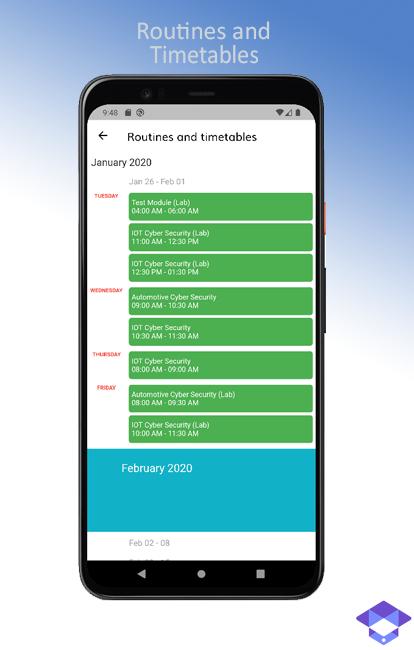This photograph features a cell phone set against a vertically oriented rectangular background. The background gradates from a rich blue in the upper right corner to a pristine white towards the bottom, with most of the blue concentrated in the upper section.

Above the cell phone, bold text reads: "Routines and Timetables, Routes, Routines, and Timetables." The phone screen displays a timetable labeled "Routines and Timetables, January 2020," detailing the schedule for January 26th through February 1st. 

Here's the detailed timetable:

**Tuesday:**
- Test Module Lab: 4 a.m. to 6 a.m.
- 101 Cyber Security Lab: 11 a.m. to 12:30 p.m.
- IoT Security Lab: 12:30 p.m. to 1:30 p.m.

**Wednesday:**
- Automotive Cyber Security: 9 a.m. to 10:30 a.m.
- IoT Security: 10:30 a.m. to 11:30 a.m.

**Thursday:**
- IoT Security: 8 a.m. to 9 a.m.

**Friday:**
- Automotive Cyber Security Lab.

The photo captures the organized layout of a detailed weekly schedule, using clear and specific typography to ensure each event is easily readable.